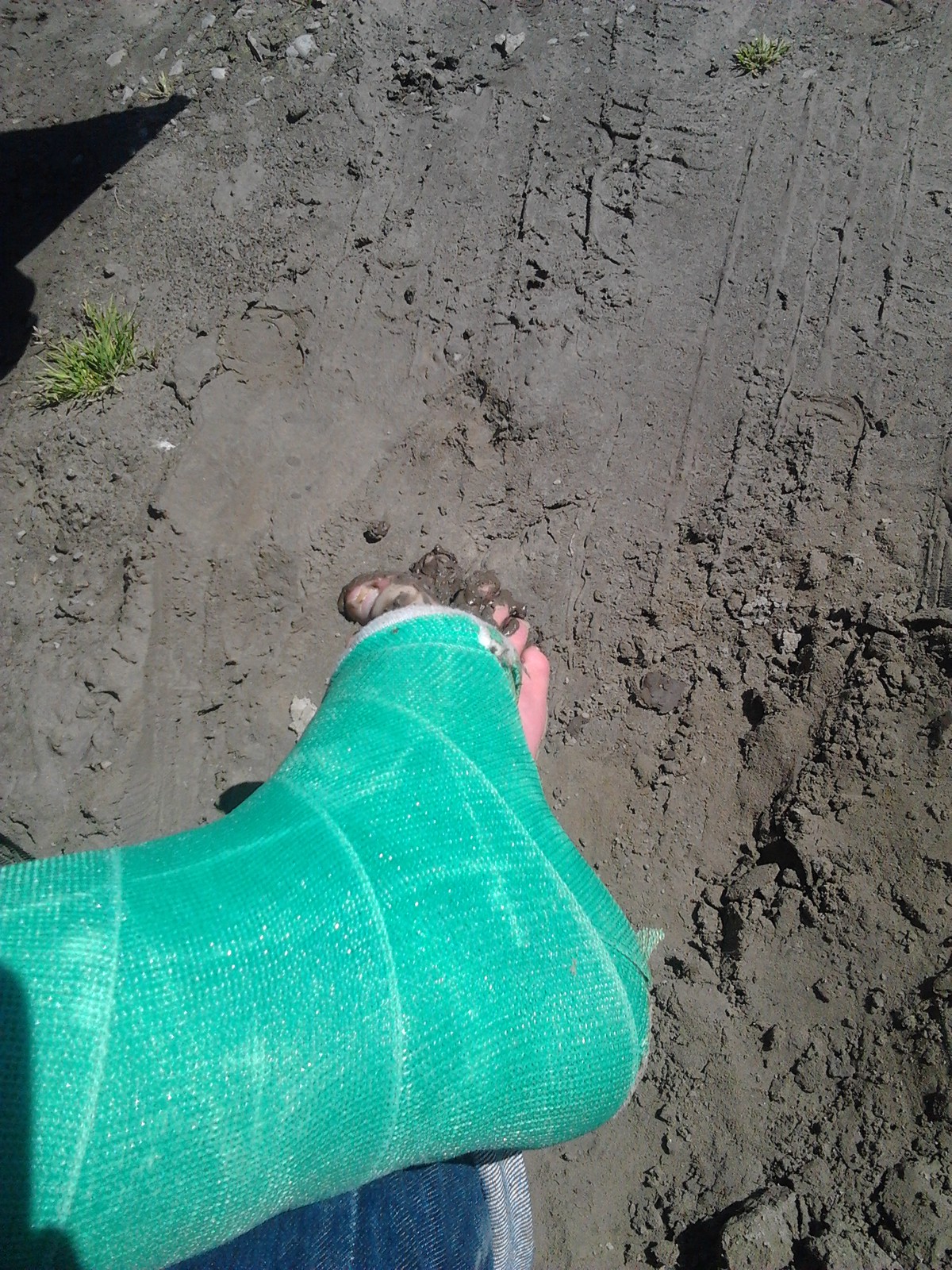In this color photograph, taken from an overhead perspective, a left foot is prominently shown digging into a sandy, muddy area. The foot, encrusted with a mix of mud and sand, is encased in a light green cast that covers the foot, ankle, and shin, leaving only the toes exposed and scrunched up in the mud. Visible just below the cast is the bottom of the person's right leg clad in dark blue denim jeans. The sparsely populated muddy ground has a patch of grass and is marked with shoe or tire treads. The well-lit image, likely taken on a sunny day, reveals a triangular shadow cast in the upper left corner.